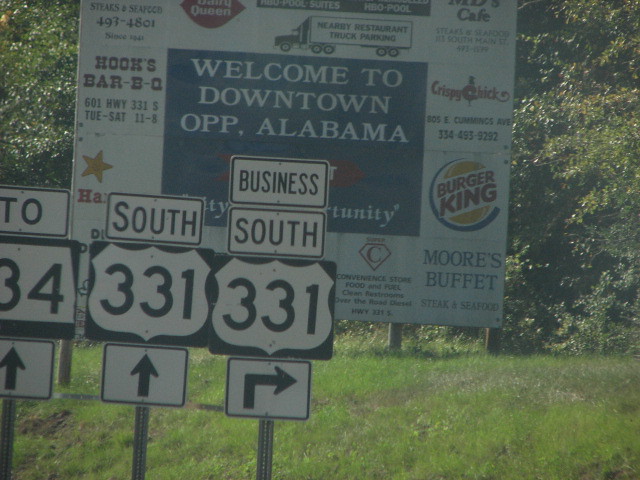The photograph captures a scene along a highway in Alabama, near the entrance to downtown Opp. The prominent Welcome to Downtown Opp, Alabama sign is surrounded by lush vegetation, which includes abundant trees and grass, indicating a verdant roadside location. In front of this large welcoming sign, there are several road signs. Two of them are clearly visible: one showing route 334 with a straight arrow, and another indicating southbound route 331, also with a straight arrow. Additionally, a third sign directs traffic towards Business South 331 to the right. The welcoming sign also lists various local dining options available in the area, such as Burger King, Hook's BBQ, and Harvey's, highlighting some of the fast-food choices for travelers entering Opp, Alabama.